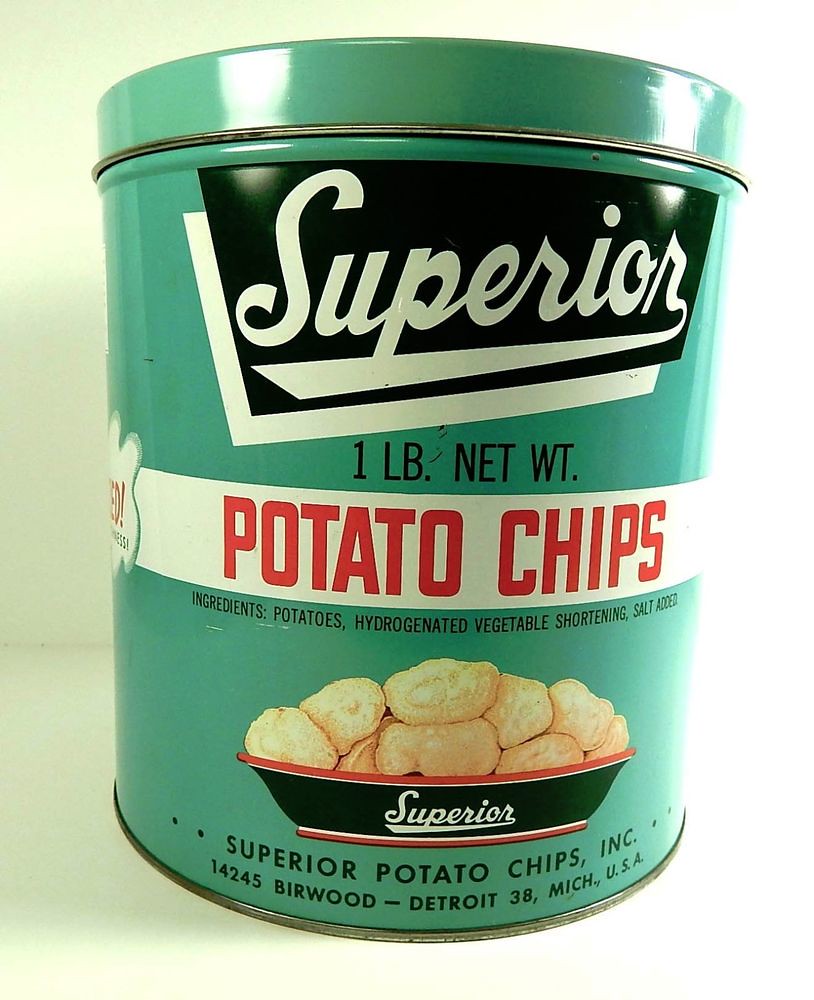The image features an old-fashioned, teal green tin container of Superior Potato Chips, set against a light grayish background. The container has a nostalgic design, reminiscent of vintage packaging. At the top, there's a black rectangular logo with white cursive lettering spelling out "Superior," and the line from the "R" underlines the entire word. Below this, "one pound net weight" is printed on the teal background. A white strip beneath this displays the words "Potato Chips" in bold red letters, and below this, another black text line lists the ingredients: "potatoes, hydrogenated vegetable shortening, salt added." Towards the bottom of the container, there's an image of a large bowl filled with thick-cut potato chips, almost resembling actual potatoes. Underneath this image, it reads "Superior Potato Chips, Incorporated, 14245 Burwood, Detroit, 38 Michigan, USA" in black text.